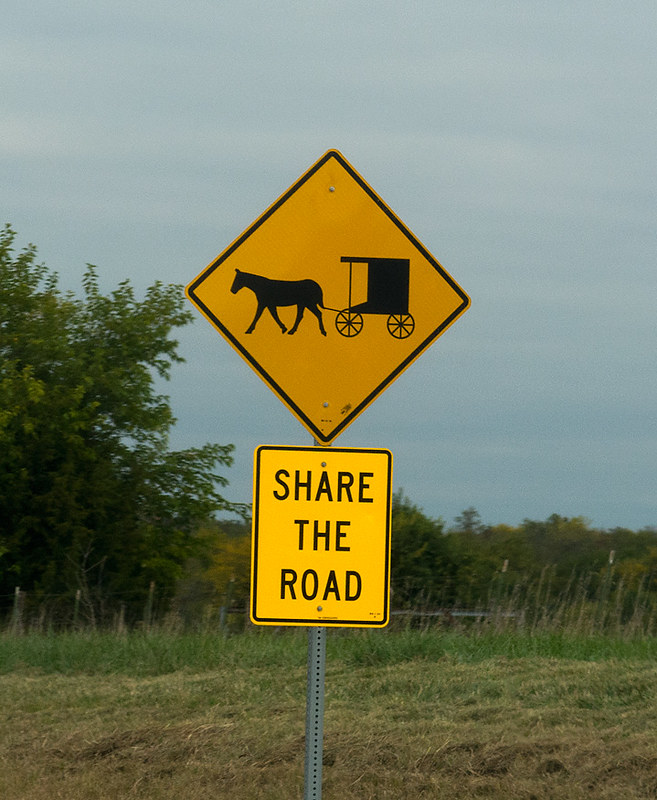A roadside sign stands prominently against a pastoral backdrop. The upper section of the sign is diamond-shaped and features a cautionary symbol: a black silhouette of an Amish horse-drawn buggy on a yellow background with a black border. Directly beneath it, a rectangular yellow sign with black text urges, "Share the Road." Both signs are mounted on a standard metal post commonly used for street signage. The background reveals a lush, grassy field transitioning from brown in the foreground to vibrant green further back. Approximately a third of the way into the image, the field gives way to a dense cluster of green bushes. Trees frame the left side of the scene, providing a natural boundary. The sky overhead exhibits a hazy blue-gray hue, lightly streaked with white, creating a tranquil and uniform canopy above the rural landscape.